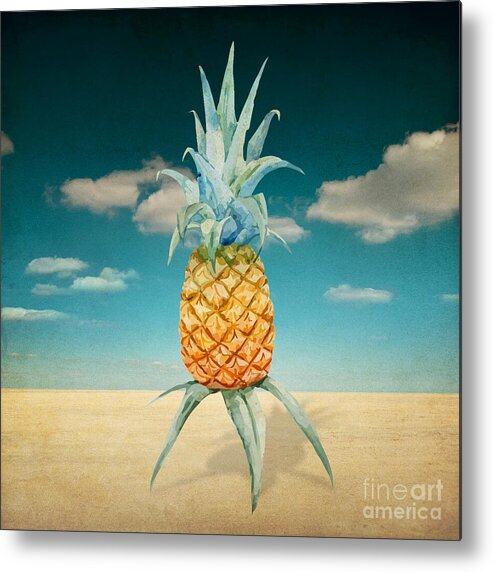This is an artistic depiction of a pineapple, prominently displayed against a vivid background. The pineapple, with its typical rough, golden-brown skin, is shown with light blue-green and light green leaves extending from the top, resembling aloe leaves. It is intriguingly positioned as if suspended just above the ground on three leaves, casting a shadow behind it that adds a fantastical element to the scene. The background features a blue sky with scattered white clouds that darken as they rise, extending to the horizon. Below the pineapple, the ground is represented by a dry, yellow field, evoking a desert landscape. This captivating image is framed within the context of a stock image, with "Fine Art America" inscribed in the bottom right corner, indicating its source.